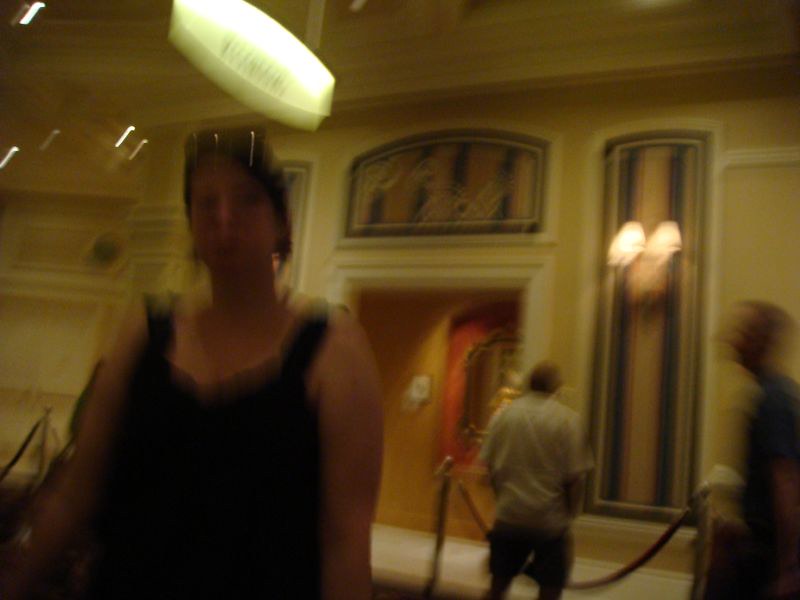In this somewhat blurry indoor photograph, likely taken in an elegant building or possibly a museum, the scene unfolds with rich detail. On the left side of the image, a woman with short, dark hair that falls just below her ears stands facing the camera, although her face is indistinct and blurred. She has sunglasses perched on her forehead and is dressed in a black tank top that stops at her midriff. The woman appears to be Caucasian.

On the opposite side, a man with short hair, possibly wearing a blue shirt, is also present but is equally blurry and indistinguishable. Positioned between the two is another individual, viewed from the back, who wears a white shirt with sleeves that reach his elbows and dark shorts. This person stands behind a stanchion barrier, the ropes supported by metallic poles, gazing at a featureless wall illuminated by a series of lights and detailed with a minimalist pattern of light and dark lines.

To the left of this central figure, there is an open doorway revealing a framed artwork within another room, which appears to be a painting. Above this doorway, there is a hint of a mural or painting adorning the higher section of the wall. The room's walls are painted a warm yellow, adorned with white molding, adding to the sense of sophistication and grandeur of the space.